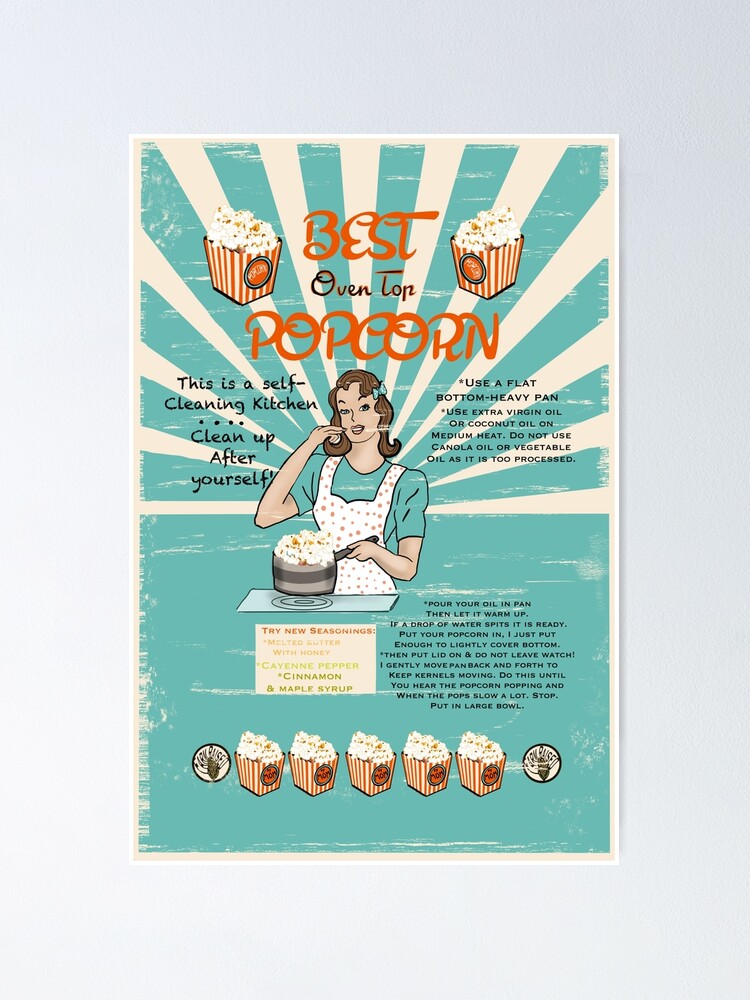This advertisement for "Best Oven-Topped Popcorn" has a vintage or retro look to it, predominantly featuring a teal color scheme with white lines radiating from the center, resembling rays of light. At the heart of the ad, a woman is prominently displayed. She is dressed in a teal shirt underneath a white apron adorned with pink polka dots, complemented by a teal bow in her brunette, shoulder-length hair, which is neatly curled under. She engages the viewer with a gesture that suggests tasting—one finger poised near her mouth—while her other hand grasps a pot over a stove. The pot, equipped with a silver lid and a long gray handle, is filled with freshly popped popcorn.

Above the woman, the bold text reads "Best Popcorn" in a vibrant mix of orange cursive and brown fonts, emphasizing the product's name. To the left of the image, black text instructs, "This is a self-cleaning kitchen. Clean up after yourself." To the right, additional cooking tips recommend using a flat-bottom heavy pan with extra virgin oil or coconut oil heated on medium, cautioning against the use of canola or vegetable oil due to their processed nature. Below this, in an off-white box, a list of seasoning suggestions includes options like melted butter with honey, cayenne pepper, cinnamon, and maple syrup. Further guidance is provided in black text, detailing the popcorn-making process—from heating the oil to agitating the kernels.

Finally, the bottom of the image is decorated with illustrations of five boxes of popcorn, reinforcing the product's branding and availability.